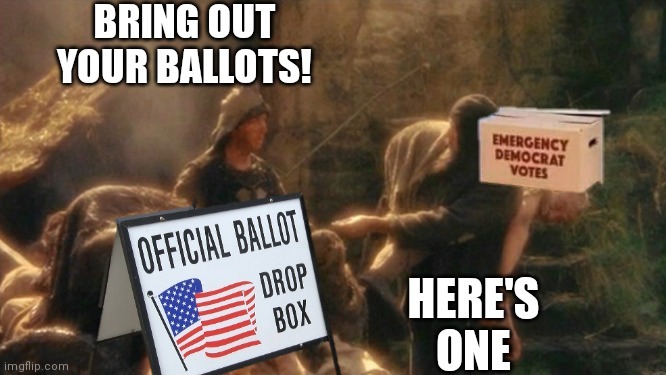This horizontal, rectangular political image prominently features a blend of text and figures with a clear right-leaning message. The image is set outdoors, possibly in a wilderness-like area. At the upper left corner, bold white all-caps letters declare "BRING OUT YOUR BALLOTS!" Below, towards the bottom left, a black-bordered white sign reads "OFFICIAL BALLOT DROPBOX" in all caps black letters, accompanied by a wavy American flag. Centered on the right, two figures stand out: one partially obscured by the official ballot sign, and the other draped in a hooded robe, extending their left hand outward. Behind this person is a white mailbox with red typography that reads "EMERGENCY DEMOCRAT VOTES." Adding to the message, at the lower right corner, white text proclaims "HERE'S ONE." The composition and elements of this visual clearly critique political practices, referencing historical contexts and invoking a nostalgic outdoor setting.